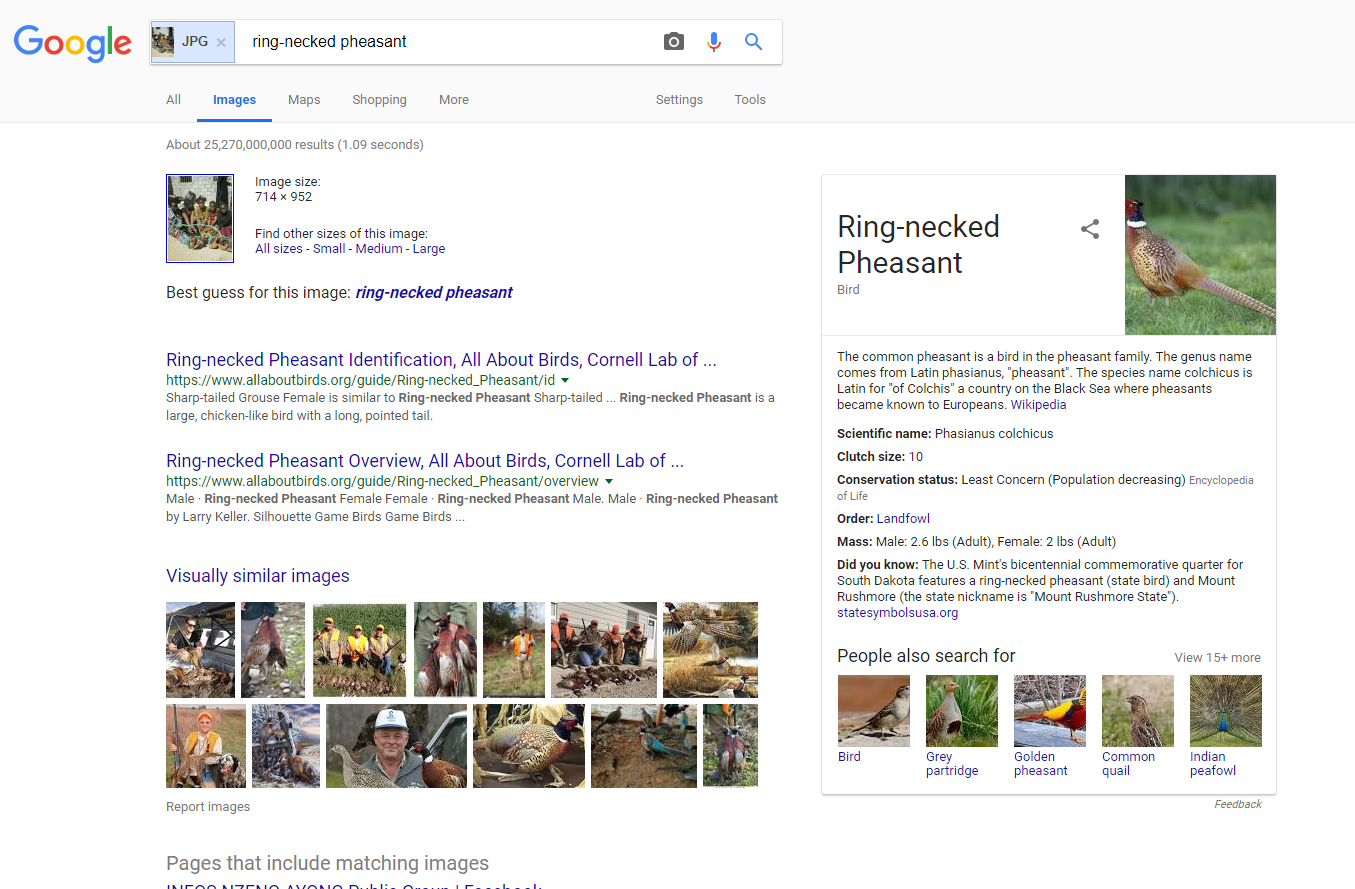This is a detailed screenshot of a Google search results page captured from a computer monitor. The primary color scheme is white, with the iconic multicolored Google logo appearing at the top left corner. 

The main search bar is prominently displayed across the top of the page. On the left side of the search bar, a blue section features a small, unclear image icon with the text "JPG" in black. To the right of this section, the search query "ring neck pheasant" is typed in black text. Further to the right, icons for a camera, microphone, and magnifying glass (search) are visible.

Beneath the search bar, the Google results menu spans horizontally. The "All" and "Images" options are listed with the latter underlined and in blue, indicating it's the current selection. "Maps," "Shopping," and "More" options appear in black, along with "Settings" and "Tools" on the far right.

The main content area starts with info about the image size, noted as 714 by 952 pixels, and a blue-outlined vertical image on the left. Below this, text invites users to "find other sizes of this image" and guesses the image as a "ring neck pheasant."

Further down, the results include web link snippets. The first link, identified in blue, is titled "Red Neck Pheasant Identification - All About Birds - Cornell Lab," and a similar URL for Cornell Lab follows.

At the bottom, there are two rows of thumbnails labeled as "visually similar images," showing around ten pictures of people with birds in various wild settings. 

In the bottom left corner, it reads "pages that include matching images."

To the right, details about the ring neck pheasant are prominently displayed. The heading "Ring Neck Pheasant" appears in black text, accompanied by an image of the bird on grassy terrain. Below, detailed information is provided, including the scientific name, clutch size, conservation status, order, mass, and a "Did You Know?" section, all in black text.

At the bottom of this section, there are five square images under the heading "People also search for," with each image hyperlinked and labeled in dark blue text as bird, gray partridge, golden pheasant, common quail, and Indian pea fowl. To the far right, it invites users to "view 15+ more."

The page concludes with a light gray "Feedback" option.